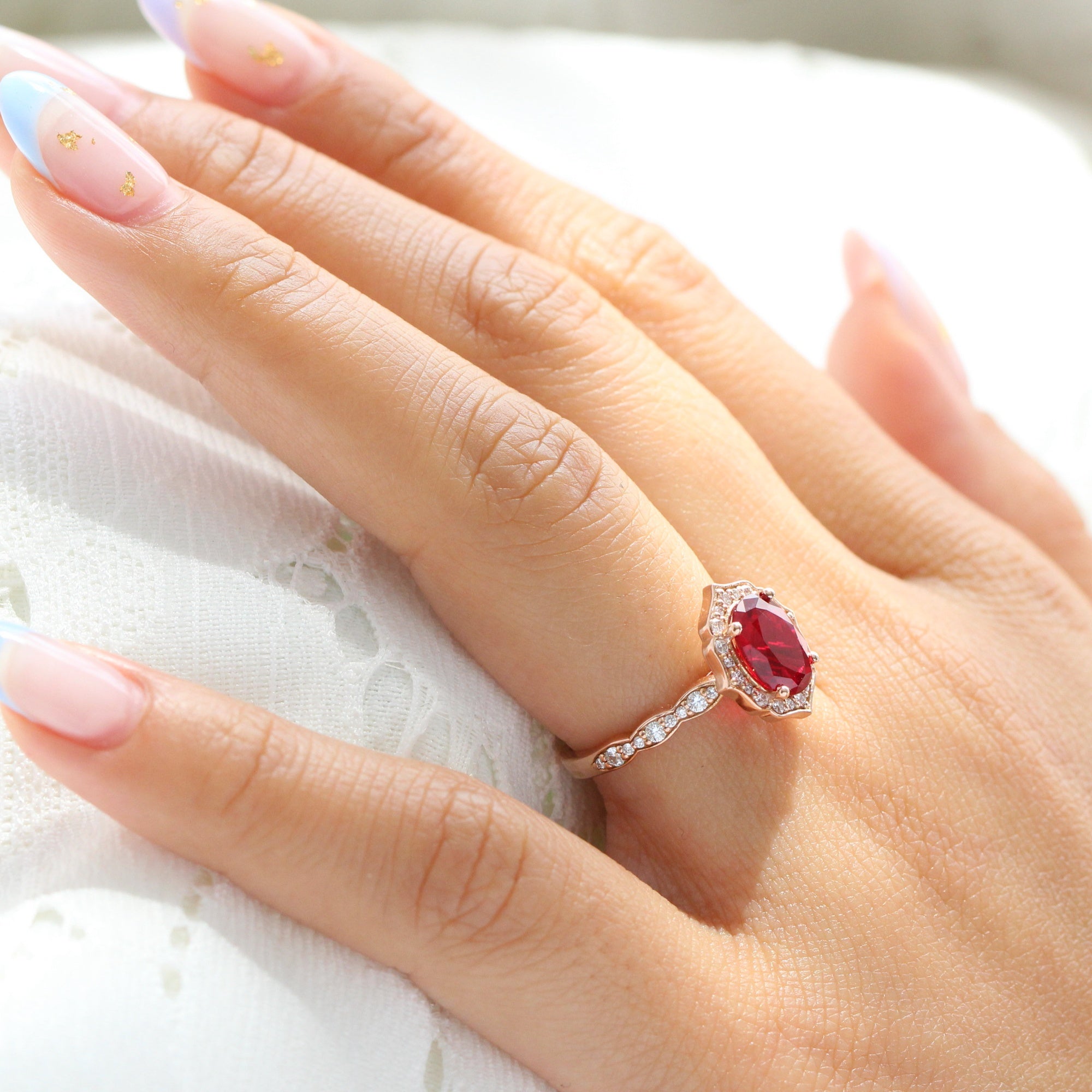This detailed up-close photograph captures the elegance of a fair-skinned woman's hand adorned with a rosy gold ring featuring an oval ruby surrounded by white diamonds. The ring's wavy band is further embellished with diamonds about three-quarters of the way around. Her nails, meticulously manicured, boast a baby pink base with light blue tips and are accented with yellow star decorations. The hand, positioned against a white eyelet fabric that resembles a lace curtain or tablecloth, is illuminated by abundant natural light, suggesting an outdoor setting. The image, shot from above and at an angle, emphasizes the vivid colors of white, pale pink, red, and bright silver against the soft backdrop. The photograph is slightly blurry on the right side due to the intense lighting.